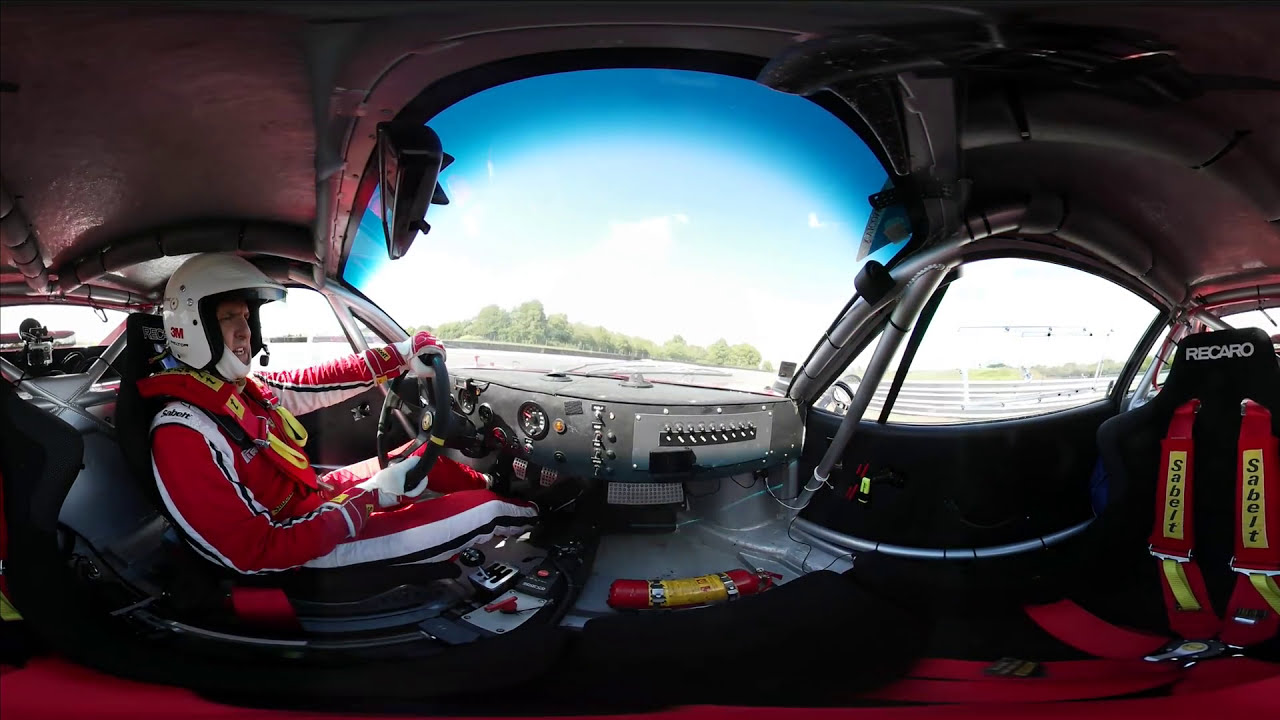The image captures the distorted interior of a race car, likely due to a fisheye lens effect. It reveals a detailed cockpit with a driver in a red and white racing jumpsuit, wearing a white helmet fitted with a microphone and strapped securely into the seat with racing harnesses displaying Ferrari symbols. The driver, a Caucasian man, is oriented towards the 2:30 position and has his hands on the steering wheel. To his left is a control panel with various switches and dials, and a fire extinguisher lying on the floor. The right side of the car features an empty seat equipped with a red seat belt marked "SABELT," indicating the brand. The car's interior roof is stylishly finished in red with smoky black details. Through the windows, one can see a bright blue sky with fluffy white clouds, a distant tree line, and a white plank-style fence, suggesting the car is positioned on a racetrack.